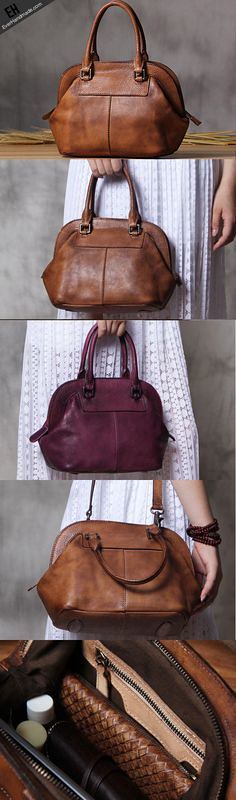This is a detailed series of five vertically-stacked photographs showcasing a stylish leather handbag from various perspectives. The top image features a dark brown leather handbag resting on a table against a gray backdrop. In the second image, the same handbag appears in a slightly lighter brown shade and is held by a person in a white dress, with only the hand and part of the dress visible. The third photograph depicts a similar handbag in a rich burgundy or dark purple color, again held by the person in the same white dress. The fourth image shows the handbag back in its lighter brown shade, now slung over the arm of the same individual, who also wears a brown rope bracelet on her wrist. The final image provides an inside view of the handbag, revealing a brown wallet and a black notepad amidst its open, light-colored interior, accompanied by small items such as a likely cosmetic product.